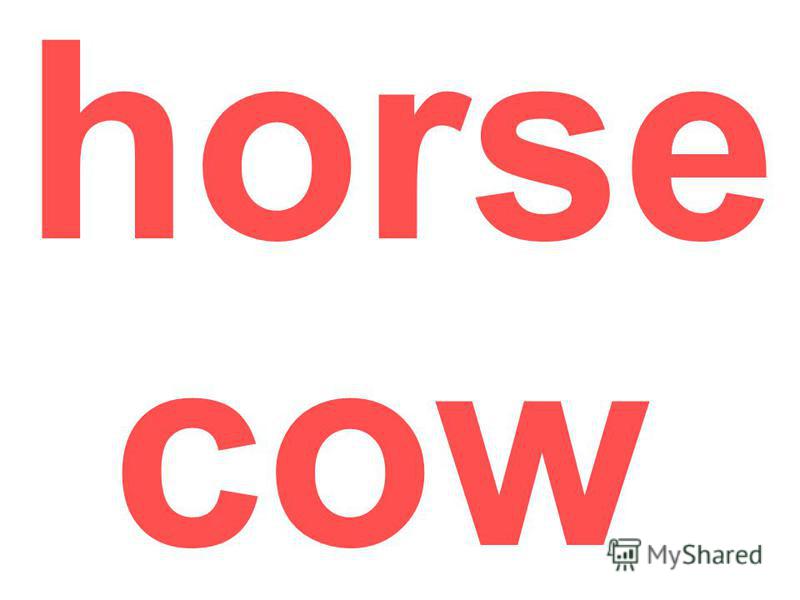This image features a graphic on a plain white background with two centrally aligned words. At the top, in a horizontally centered position, the word "horse" is displayed in a youthful, block-style font with small lowercase letters, rendered in a pale, darkish pinkish-red color. This word occupies roughly the top 20% of the image. Directly beneath "horse," after a similar-sized gap, the word "cow" appears in the same whimsical lowercase font and color, taking up a significant portion of the image's middle section. The overall presentation evokes a light-hearted and child-friendly feel.

In the lower right-hand corner, just below "cow," there is a small, intricate sketch-like company logo. This logo resembles an easel with three legs, a framed picture mounted on a stand, and a light positioned above it. Next to this logo, the phrase "My Shared" is inscribed with a distinct capitalization pattern: "M" for "My" and "S" for "Shared," with the rest of the letters in lowercase (MyShared). This text completes the playful yet structured design of the graphic.